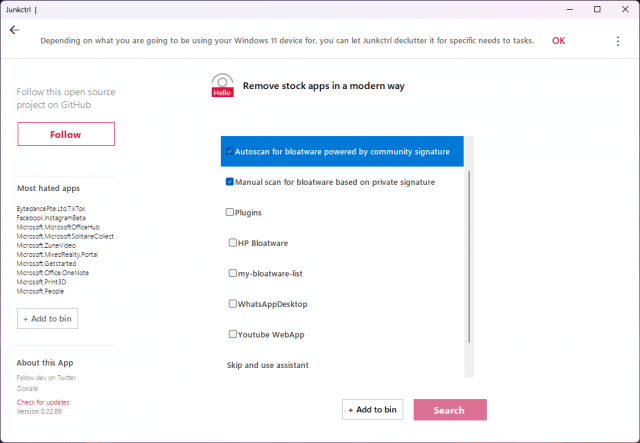The image is a screen capture of a web page featuring the Junk CTRL interface. The top left corner prominently displays the title "Junk CTRL" with a subtitle "Junk Control" within a gray bezel. Adjacent to the title, on the right side of the bezel, there are controls for window management: a minus symbol for minimizing, a square symbol for expanding, and an "X" for closing the window.

Within a rectangular white bezel below, there is a black arrow on the left and a hot pink "OK" (spelled "OK", not "OKAY") on the right. The area also contains black text stating: "Depending on what you are going to be using your Windows 11 device for, you can let Junk CTRL declutter it for specific needs to task."

In the middle section of the page, there is an icon of a person over a circle with a red rectangle displaying white text that reads "Hello." To the right of this icon, it says "Remove stock app in a modern way."

Further down, a dark blue bezel encloses a square that reads "Automation for Bioware powered by Community Signature." Below this, a blue check mark is next to another square with the text "Mutual scan for Bioware based on Private Signature."

Additionally, there are several unchecked gray squares aligned vertically with labels including: "HP Bloatware," "My-Bloatware-List," "WhatsApp Desktop," "Youtube Webpage," and "Skip and Use Assistant."

On the left side of the interface, there is a notation that reads "This is an open source project on GitHub." Below this notation is a red rectangle with red text in the center that says "Follow."